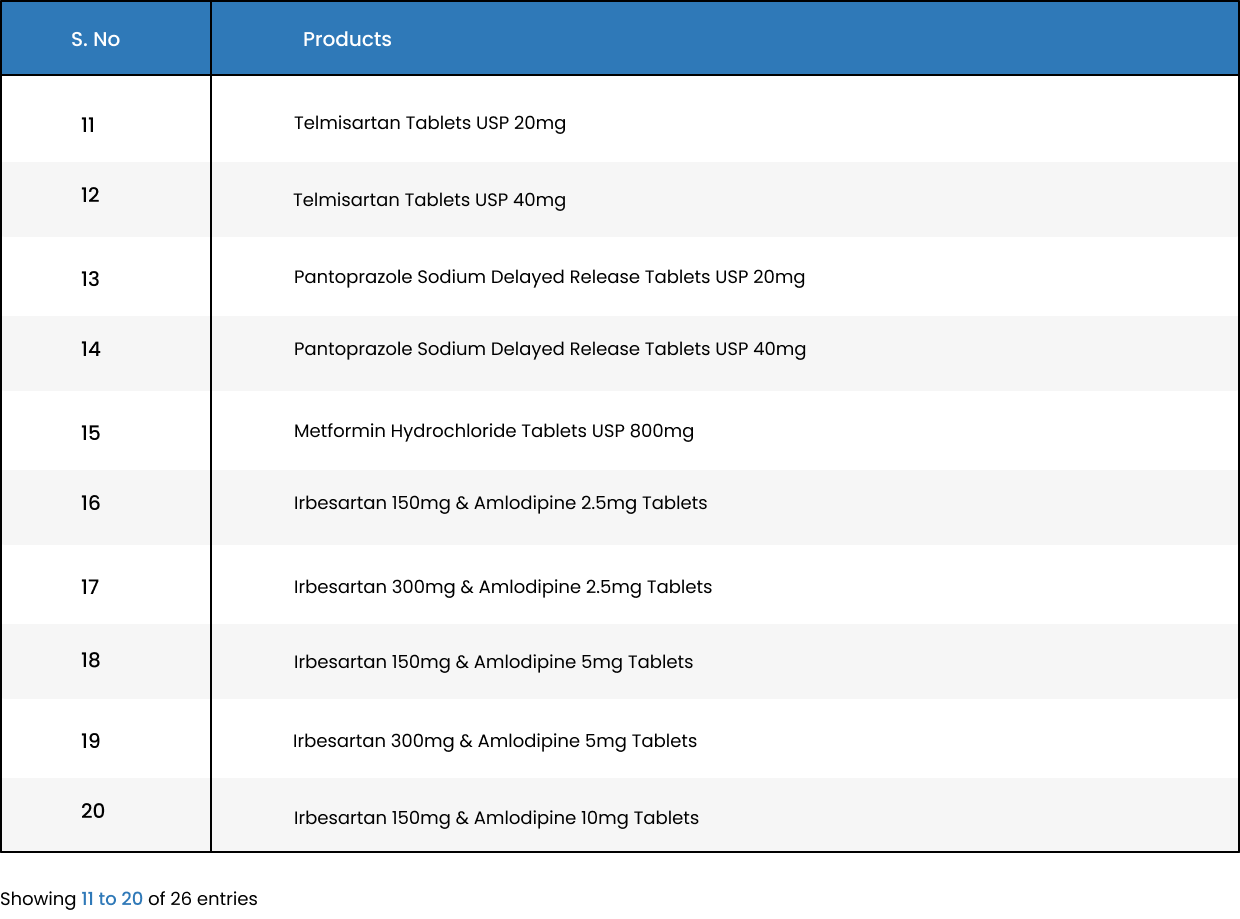The image displays a website with a structured table featuring two columns: "S.NO" (Serial Number) and "Products." Both column headers are presented in blue bars with white text. The table lists various pharmaceutical products, each associated with a serial number from 11 to 20. 

- **Serial Number 11**: Tels Martin Tablets USP 20mg
- **Serial Number 12**: Telmarcetin Tablets USP 40mg
- **Serial Number 13**: Pantoprazol Sodium Delayed Release Tablets USP 20mg
- **Serial Number 14**: Pantoprazol Sodium Delayed Release Tablets USP 40mg
- **Serial Number 15**: Malfortum Hydrochloride Tablets USP 800mg
- **Serial Number 16**: Irbesartan 150mg and Amlodipine 2.5mg
- **Serial Number 17**: Irbesartan 300mg and Amlodipine 2.5mg
- **Serial Number 18**: Irbesartan 150mg and Amlodipine 5mg
- **Serial Number 19**: Irbesartan 300mg and Amlodipine 5mg
- **Serial Number 20**: Irbesartan 150mg and Amlodipine 10mg

At the bottom of the table, a note in blue text reads, "Showing 11 to 20 of 26 entries."